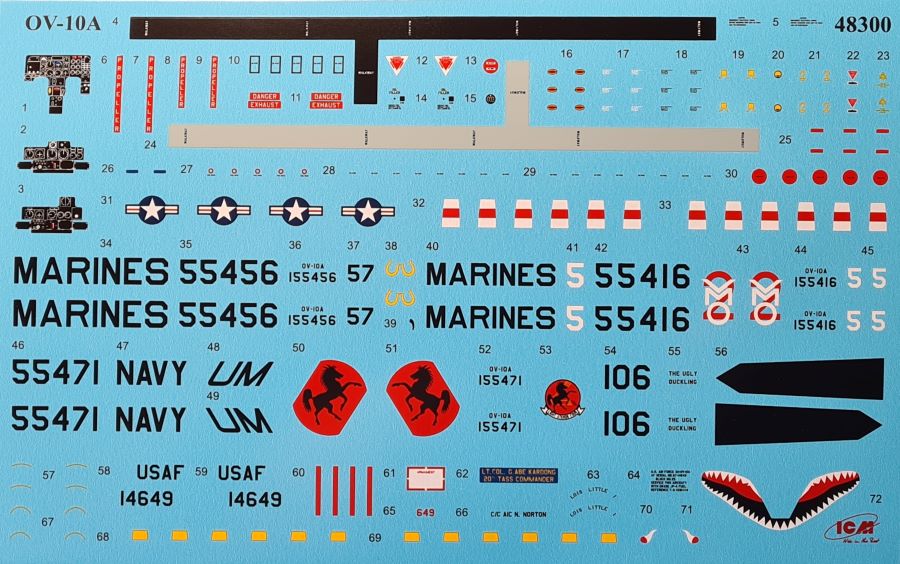This image is a detailed decal sheet for a model kit, likely representing military equipment such as a jet or a boat. The background is a turquoise light blue, with two horizontal bars at the top—one black and one gray. These bars contain various symbols and numbers, with the black bar featuring a small downward protrusion just left of its center. 

Prominently displayed in the center are repeating phrases: "Marines 55456" and "Marines 55416," each followed by a smaller line stating the same. Below these, "55471 Navy" is featured, accompanied by a detailed dog tag depicting a Pegasus or horse. Further down, a line marked "USAF 14649" is highlighted with four red lines and accompanied by smaller icons.

Additional symbols and numbers are scattered throughout the sheet, with several red and blue circles featuring white stars, dotted lines, and other military insignias. A prominent emblem in the bottom right corner showcases jagged shark teeth, hinting at its aviation or maritime application. This detailed labeling provides comprehensive embellishments to complete the look of the plastic model once assembled.